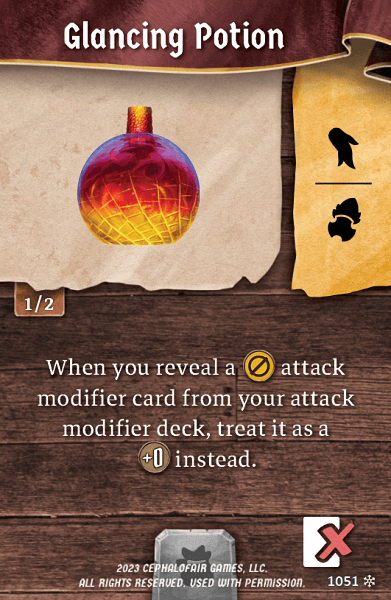This is a detailed screenshot from a game interface, showcasing an item titled "Glancing Potion" prominently at the top. The potion icon is situated in the top left corner, depicted as an apothecary bottle with visible damage and cracks. The potion displays a radiant yellow to red gradient, enhancing its visual appeal. Below the potion, there is accompanying text that reads: "When you reveal an attack modifier card from your attack modifier deck, treat it as a +0 instead." Adjacent to the word "attack" is a yellow circle featuring a cross-out symbol inside it. Adding to the aesthetic, the background under the text resembles parchment paper, laid over what appears to be a wooden table. Above the potion's title, "Glancing Potion," there is a red fabric material accented with a golden border, giving the scene an antiquated charm. For additional context, a white card with a red X is visible in the bottom right corner of the image.